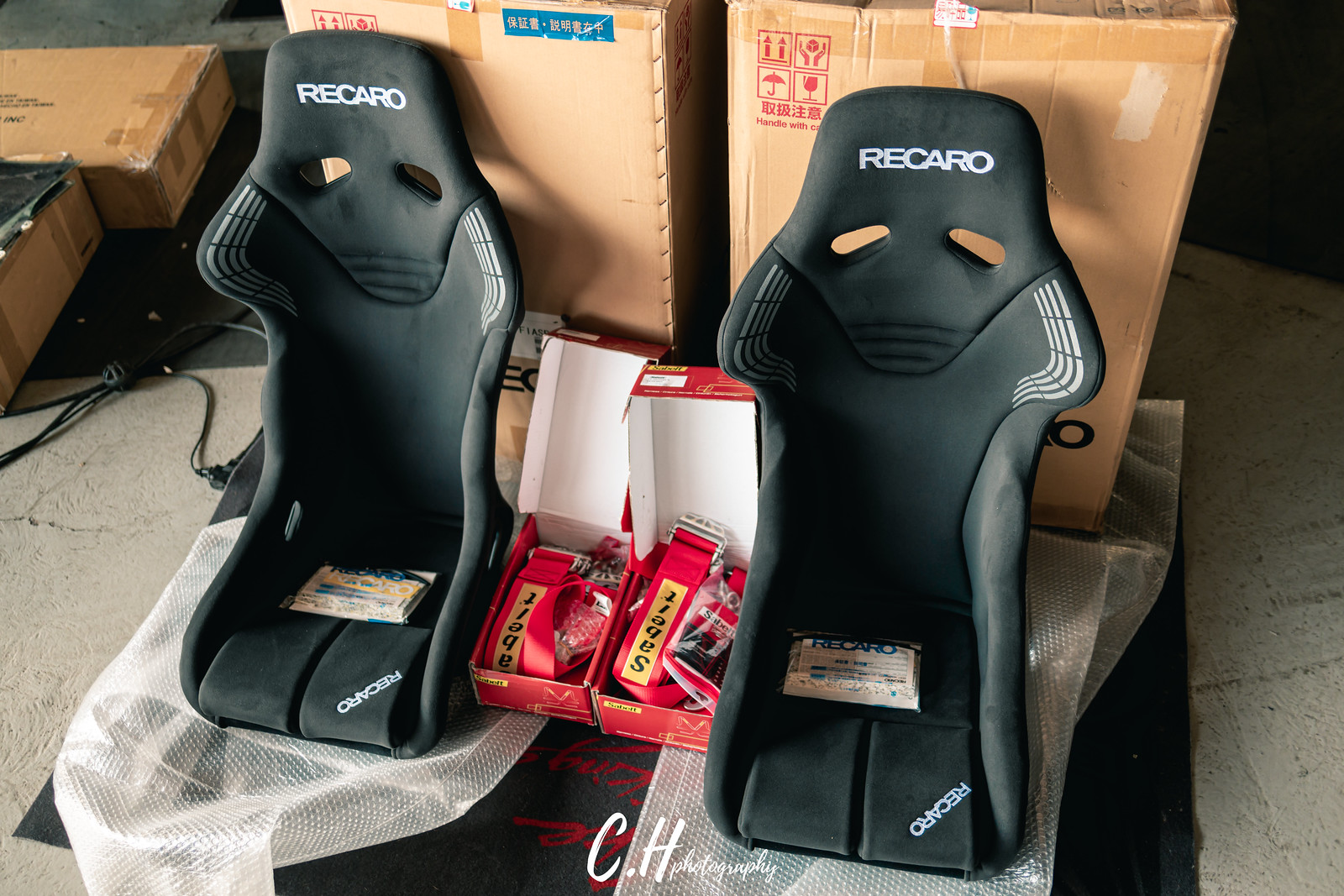The image is a detailed color photograph, oriented in landscape, showcasing two identical black Recaro vehicular seats. These seats, possibly designed for high-performance racing or child safety, feature a foam rubber design with widened shoulder backings and narrow profiles. Each seat prominently displays the Recaro brand name on the headrest area. The seats are placed side by side on a concrete floor, resting on pieces of white bubble wrap, and propped against large cardboard boxes likely used for shipping. Between the seats are two open red boxes, revealing thick red canvas seat belts. Additional cardboard boxes are visible in the background, contributing to the setting of what appears to be a storage or packaging area. The image is marked with the credit "CH Photography" at the bottom, highlighting its professional representation.